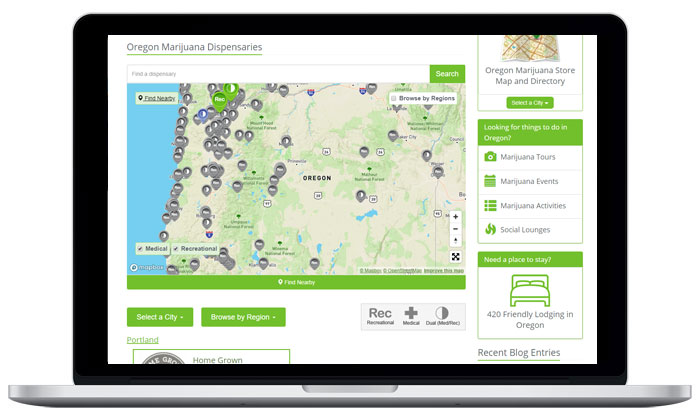The image shows a silver laptop viewed from the side, revealing its sleek keyboard design. The laptop's screen, encased in a black border, displays a detailed interface. The top part of the screen is gray, prominently featuring the phrase "all the time in one dispensary," underlined in green. Below it is what appears to be a map distinguishing water on the left in blue and land on the right in beige and green.

Text elements on the map are in black, including labels such as "recreational," "medical," "nearby," and "browsed by region." However, the specific names of streets are not visible. At the bottom of the screen, the options to "search" and "select a city" are displayed in white text on green background rectangles, alongside "browsed by region." 

The right side of the screen lists categories like "marijuana tours," "marijuana events," and "marijuana activities." Additionally, there are notes in white text such as "need a place to stay" accompanied by a green bed icon, and "420 Friendly Lodging in Oregon," all in black text. Lastly, the phrase "recent block entries" is also noted in black. The interface appears to be an interactive map related to marijuana dispensaries and activities in Oregon.